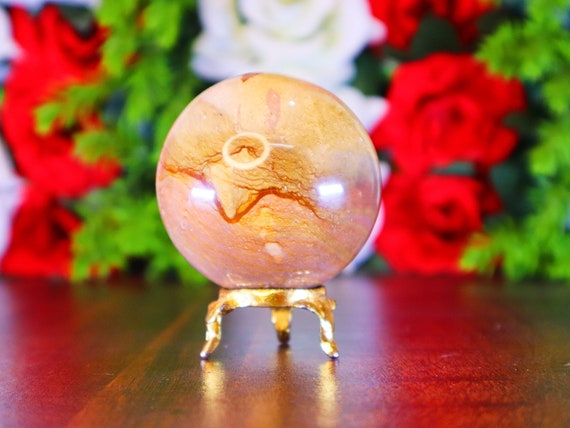The image depicts a striking piece of art set against a well-lit backdrop. The centerpiece is a shiny, orb-like object, which appears to be a beautifully crafted marble or a glass globe. The orb boasts a smooth texture with a mesmerizing blend of yellowish, pinkish, and brown hues, accentuated by bold red and orange lines that swirl around it, reminiscent of planetary patterns. This exquisite artifact is elevated on a small, golden metallic stand with three legs, lifting it two to three inches off a polished wooden table. In the background, a collection of vibrant red and white roses, accompanied by green leaves, adds to the visual appeal, though they appear slightly blurred. The careful lighting highlights the orb's glossy surface and the rich texture of the wooden table, emphasizing the artifact's display.